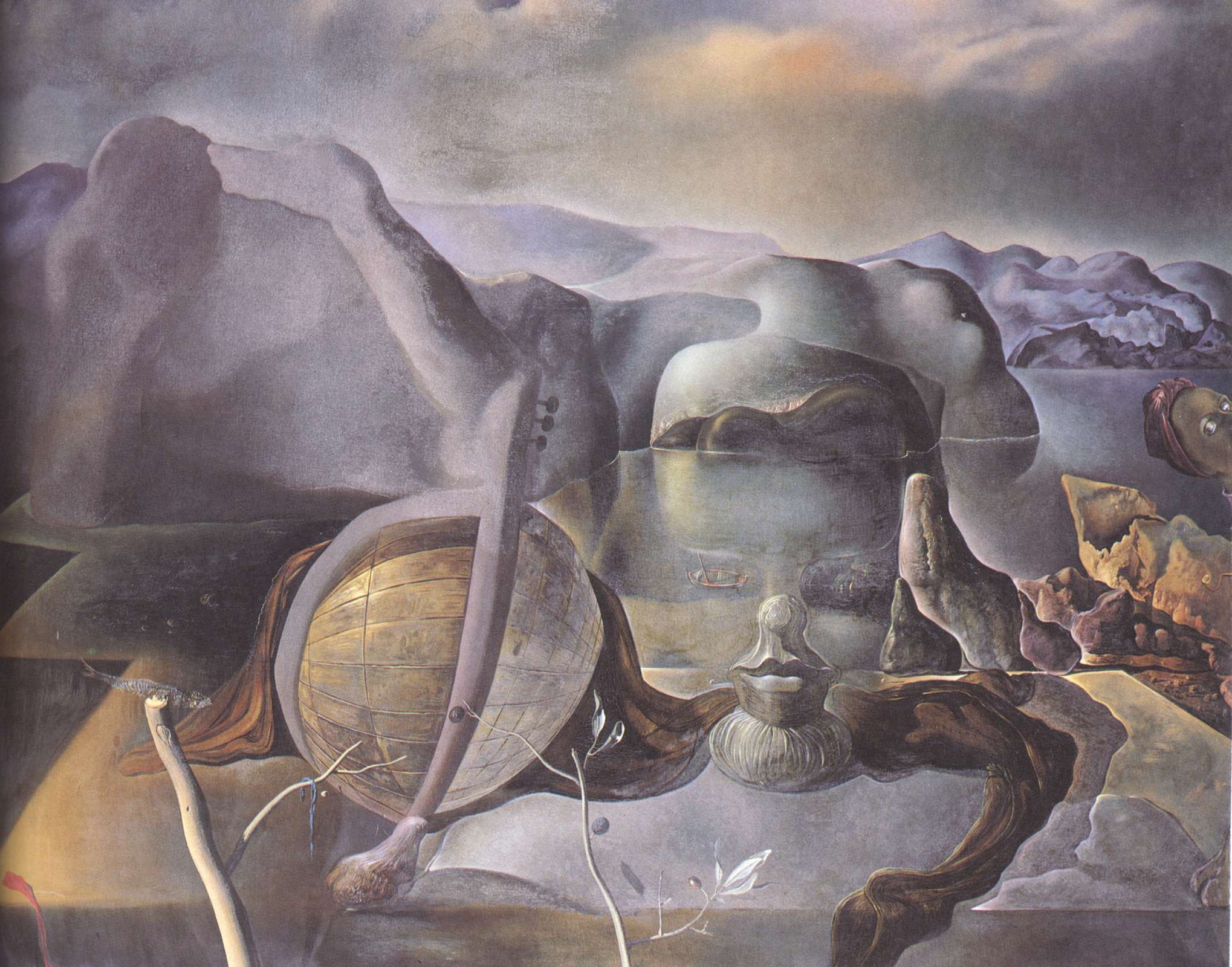The image is a surrealist painting, reminiscent of Salvador Dali's style, depicting an outdoor scene in the middle of the day. The upper part of the painting shows a cloud-filled sky. The dominant color palette ranges from black, white, and gray to splashes of gold, yellow, pink, brown, and light purple. In the chaotic and scattered composition, various objects blend and overlap, making it difficult to distinguish individual elements. 

At the bottom of the painting, there appears to be a melting globe, a stick, and a bottle-shaped object resembling facial features like lips and a nose. A piece of brown fabric is draped over a tabletop, next to a fading face of a man that merges with the gray-toned background of hills or mountain-like forms. These hills give a fleshy, body part impression, resembling shoulders and arms, creating an illusion of a larger human face with hair, lips, and eyes at the painting's center.

To the right side of the image, another face appears, with only the eyes and wrapped in a red head wrap, peeking from the edge. No text is present in the image, allowing the viewer's eyes to explore the intriguing and dreamlike elements that comprise this vivid, surreal landscape.